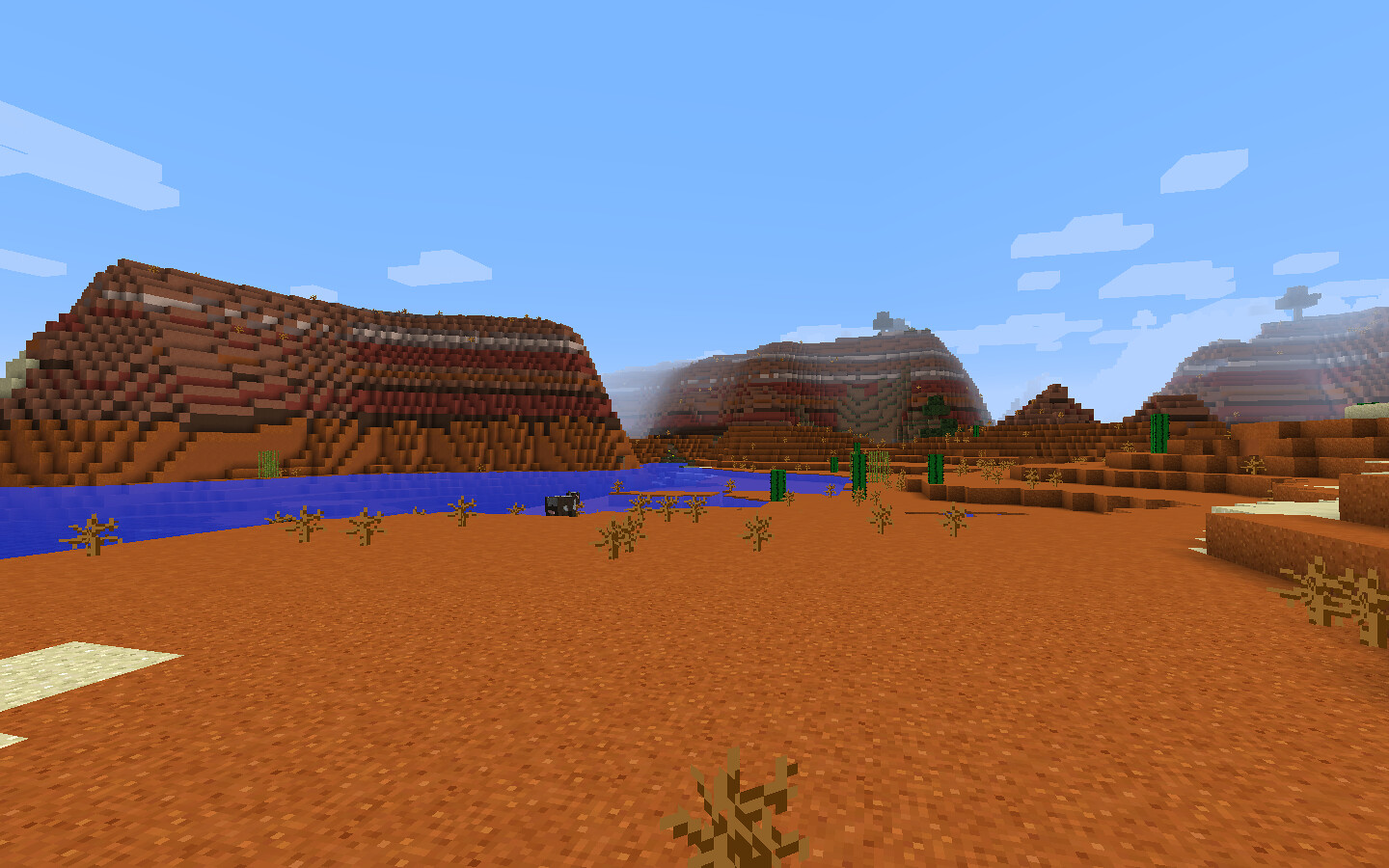The image depicts an expansive open field with a desert-like ambiance, reminiscent of a Minecraft video game scene. In the distance, there are three prominent mountains and a smaller, pyramid-shaped formation, all constructed from large, blocky components in hues of red, brown, white, and green. The mountains appear jagged and irregular, emphasizing their brick-like composition. To the left of the image, a patch of blue water contrasts against the sandy terrain, which is sparsely dotted with small green plants. Scattered light-colored blocks suggest the presence of stone embedded in the ground, further adding to the textured landscape.